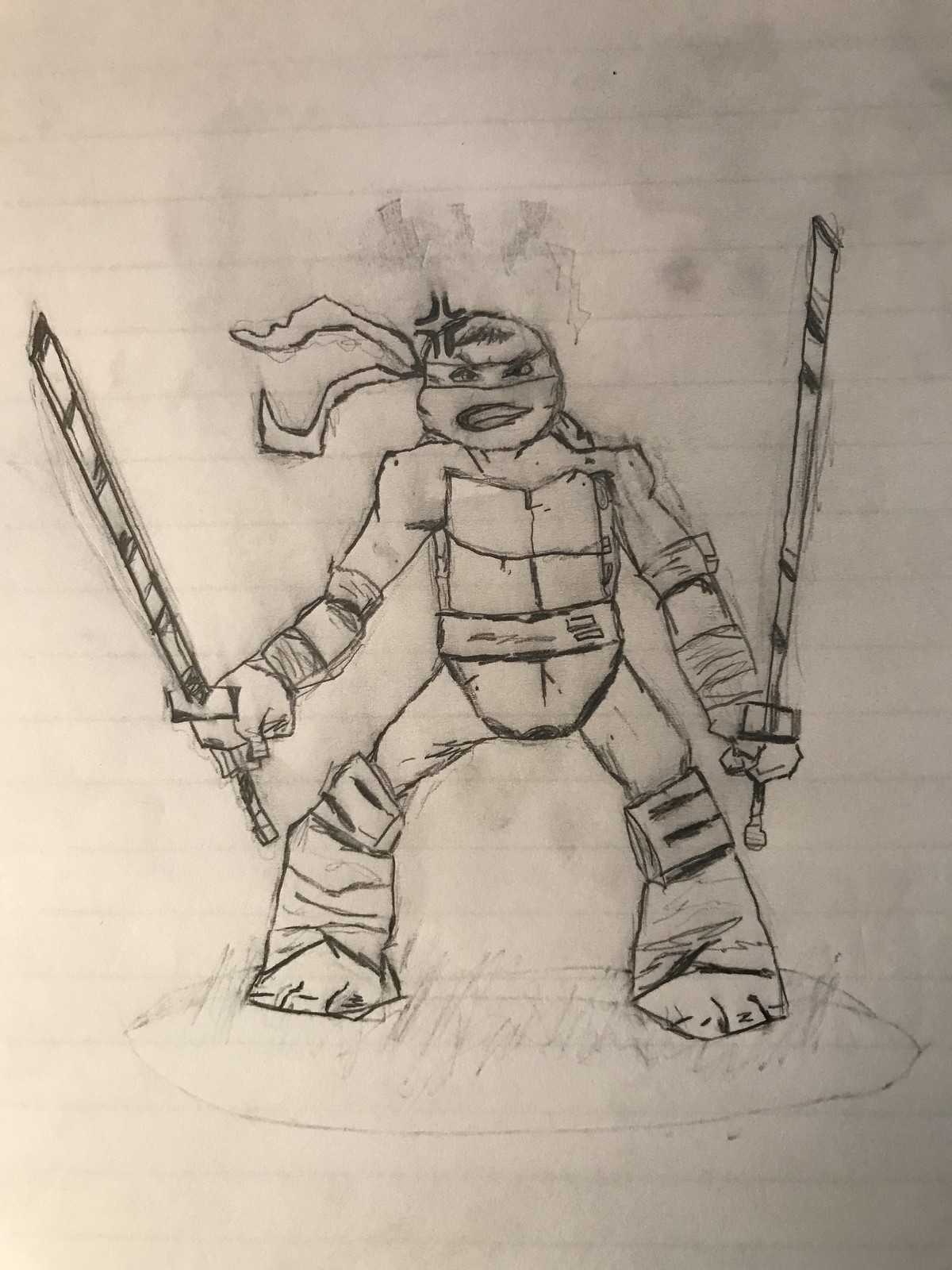The image is a detailed, black-and-white pencil drawing of a Teenage Mutant Ninja Turtle, centered on a piece of notebook paper with blue horizontal lines. The Turtle, depicted in a battle-ready stance, stands firmly on an elongated oval shape that stretches almost the entire width of the page, approximately two inches from the bottom edge.

The Turtle, facing directly forward, wields two long katana swords—one held straight up and the other slightly angled to the left. Its arms extend downwards and diagonally outwards, gripping the swords firmly. Detailed features include a circular head adorned with a bandana tied around the eyes, its ends flowing to the left as if caught in the wind. The Turtle's facial expression is fierce, with a grimace emphasizing an open mouth skewed more to the left.

Additional elements in the drawing reveal the Turtle's muscular build, with distinct elbow pads on its arms and knee guards protecting its legs, which are spread slightly apart and angled outward before ending in feet with defined toes. A shell is visible on the front, belted around the waist. Minor smudges of gray can be seen throughout the drawing, possibly from the artist's hand or as intentional shading to suggest clouds or smoke. This adds a subtle touch to the overall dynamic and action-ready appearance of the character.